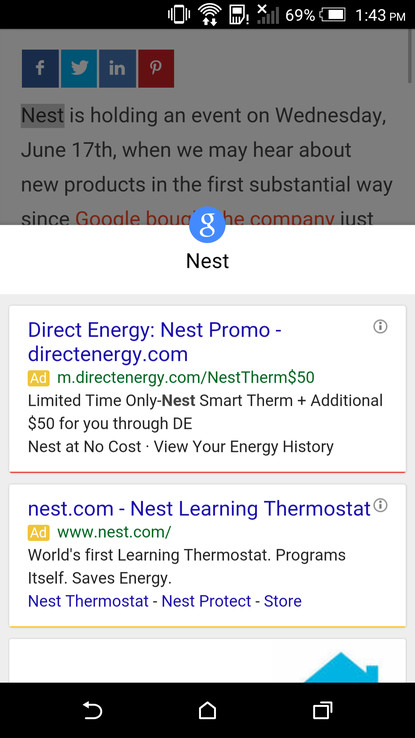The top portion of the image showcases a black status bar from a cell phone, displaying a battery level of 69%, the time which is 1:43 PM, and other typical signal indicators. Just below this, in a grayed-out area, there are several app icons: a blue square with a lowercase "f" for Facebook, a light blue square with a bird for Twitter, a blue square with "in" for LinkedIn, and a red square with a "P" for Pinterest.

Following these icons, there is a gray square containing the word "Nest" in white text. Underneath, a red-highlighted notification reads: "Nest is holding an event on Wednesday, June 17th, where we may hear about new products in the first substantial way since Google acquired the company."

Below this notification, there's a blue circle with a lowercase "g" representing Google. Further down, the word "Nest" appears again, accompanied by another gray square that contains the text: "Direct Energy Nest Promo available at directenergy.com/NestTherm $50."

The next gray square states: "Nest.com - Nest Learning Thermostat: World's first learning thermostat programs itself." Following that, three clickable blue links are labeled: "Nest Thermostat," "Nest Protect," and "Store."